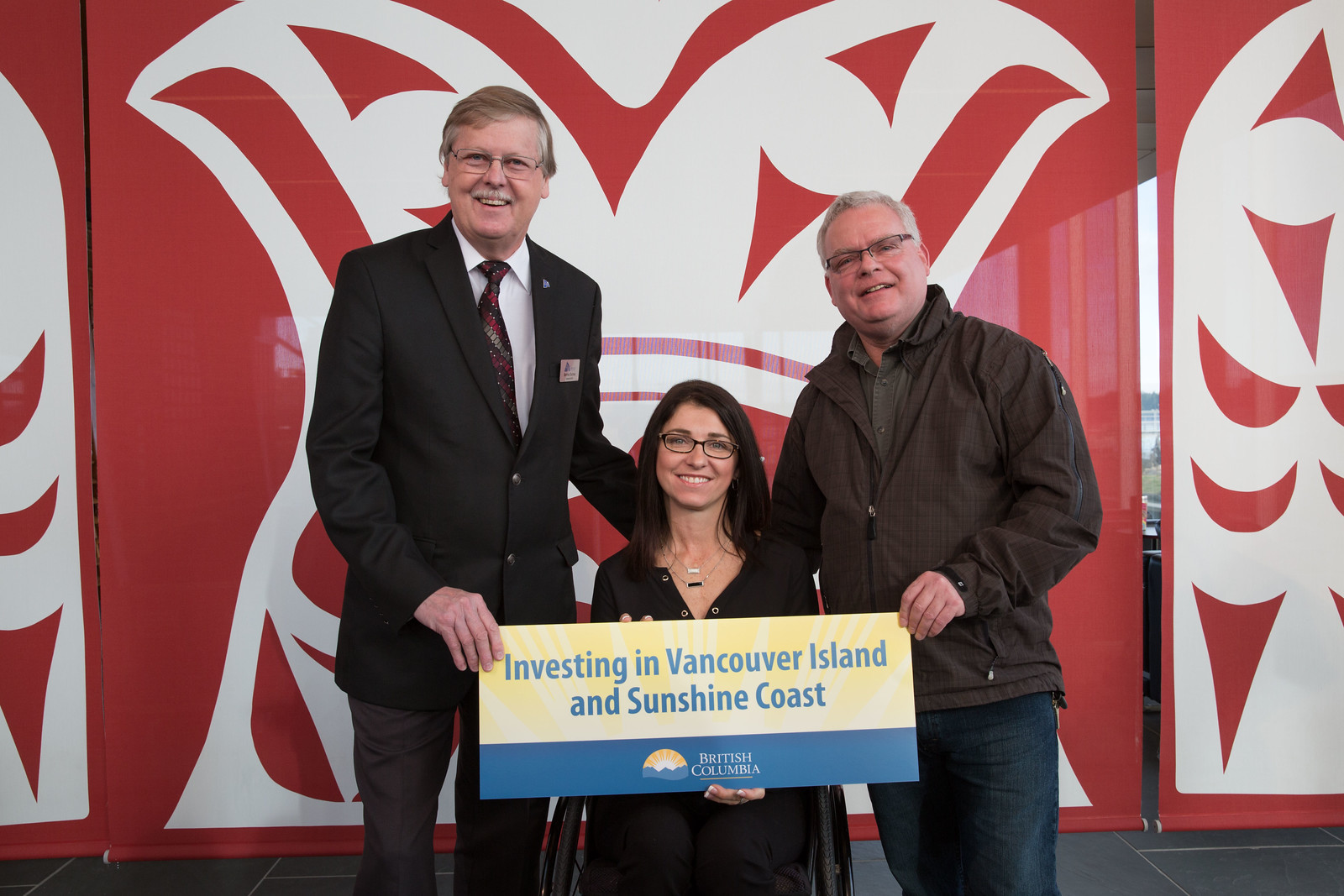The photograph captures two elderly Caucasian men and a woman in a wheelchair standing in front of a red and white banner featuring a geometric design. The woman, dressed in black, is smiling warmly as she holds a placard that reads "Investing in Vancouver Island and Sunshine Coast, British Columbia." Both men are wearing glasses and are positioned on either side of the woman, each with one hand behind her and the other hand on the placard. The man on the left is dressed in a suit and tie, while the man on the right wears a brown windbreaker. The scene appears formal, possibly depicting the presentation of an award or grant in a setting that emphasizes community investment.